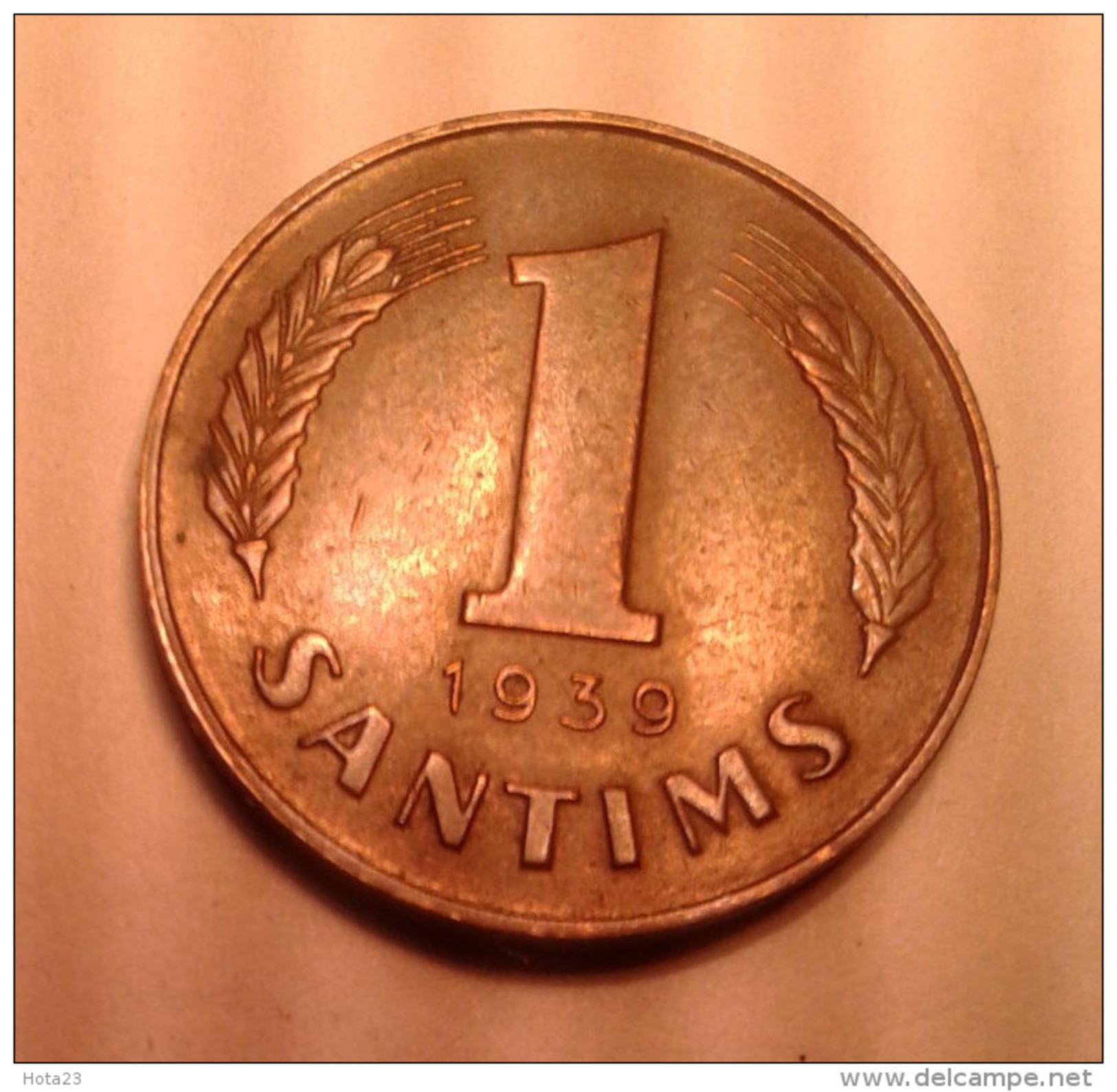The image is a close-up photograph of a copper-colored coin, centrally positioned on a pinkish background and slightly tilted to the right. The coin features two curving wheat stalks; the one on the left curves to the right, and the one on the right curves to the left. They have lines extending from their tops, almost reaching the top of a large number "1" prominently placed in the middle. Below the "1" is the date "1939," and along the bottom edge of the coin is the word "SANTIMS," with the letters starting from the base of the wheat stalk on the left and reaching the base of the wheat stalk on the right. The coin appears to be either bronze or copper-colored. In the bottom right corner of the image, there's a website URL, www.delcampi.net, and some indistinct writing, possibly including the number "23," is visible in the bottom left corner. The presented coin is likely a lower denomination currency, given its relatively simple design.